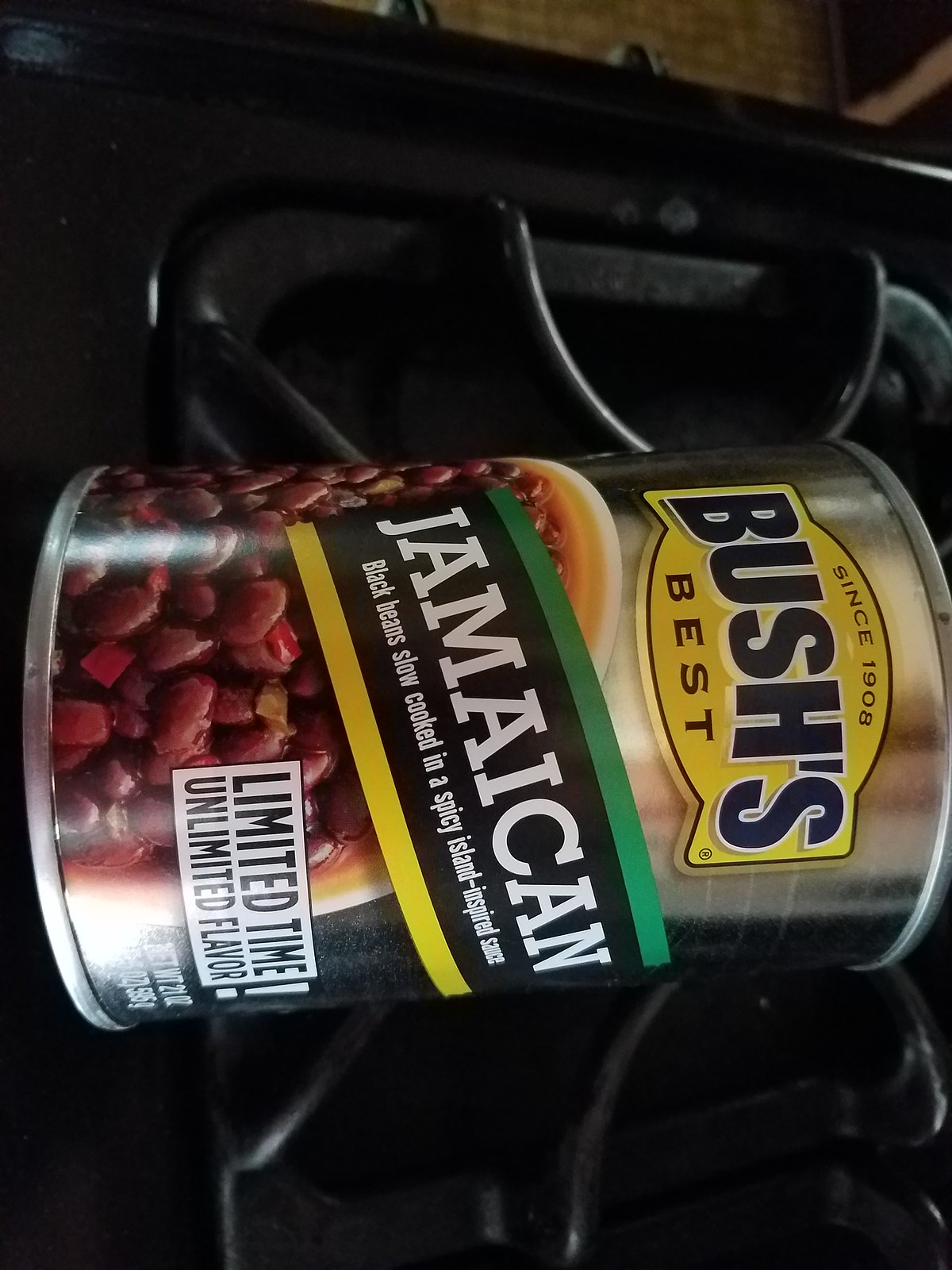This close-up rectangular image features a can of "Bush's Best Jamaican Black Beans," resting on its side with the label facing left. The can is silver, adorned with a yellow label showcasing the brand name "Bush's" in bold black text. Below the brand name, there's an enticing image of a bowl filled with black beans luxuriously immersed in a rich, brown sauce. Prominently displayed across the lower right corner, in bold white text, is a message stating, "Limited Time Unlimited Flavor." A vibrant banner spanning the front of the can, displaying the Jamaican colors of green, black, and yellow, reads "JAMAICAN" in capitalized white letters, emphasizing the island-inspired, spicy flavor of the beans.